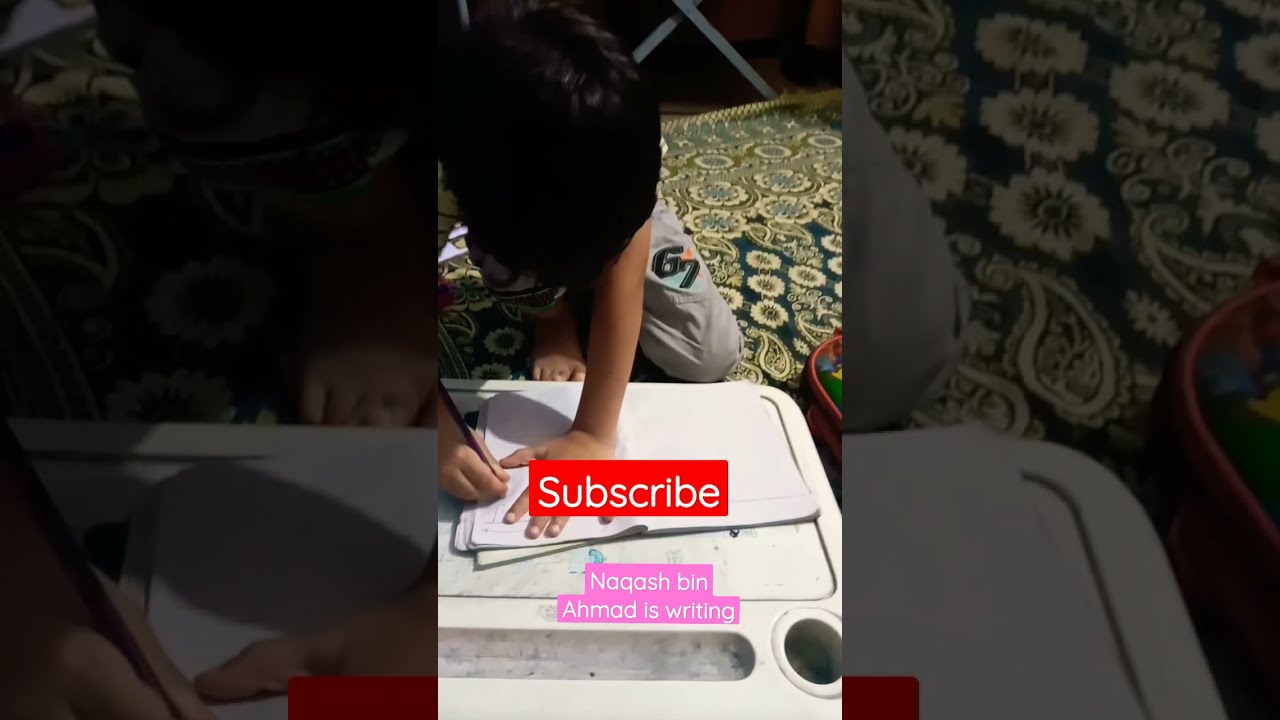The image captures a young boy with dark hair and caramel skin, sitting on a predominantly blue and yellow patterned rug. He is dressed in gray pants that feature a blue number '67' accented with a bit of orange. The boy is engaged in an activity, tracing the outline of his left hand on a white piece of paper placed on a white stand. The scene seems to take place in a domestic setting, with the boy slightly off-center towards the left. Above the scene, superimposed text includes a red rectangle with white lettering that reads "subscribe," followed by white text on a pink background stating "Nakash bin Ahmad is writing." This image appears to be a promotional screenshot likely intended for social media or a video, displaying the child's hand-tracing activity on a vertically-oriented phone screen, with the background artfully merged into a larger rectangular format.